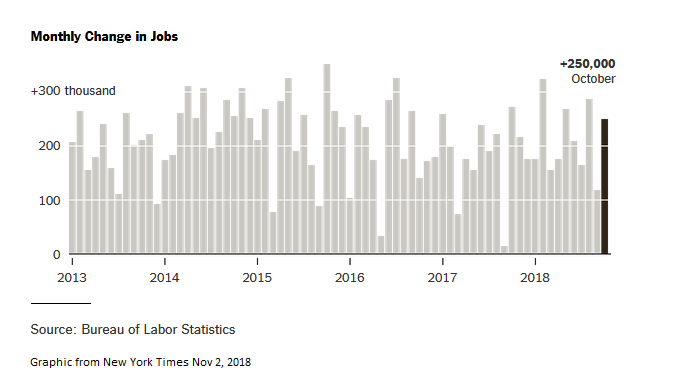The image is a detailed bar chart titled "Monthly Change in Jobs" in bold black print located at the upper left corner. The vertical axis ranges from 0 to 300,000 jobs, while the horizontal axis spans from the year 2013 to 2018. Notably, the top right corner of the chart highlights a significant job increase of over 250,000 in October. The bars on the chart are primarily light gray, depicting fluctuations in job numbers across the years, with a single distinctive black bar at the extreme right representing the October data point. At the bottom, the source of the data is credited to the Bureau of Labor Statistics, and the graphic is attributed to the New York Times, dated November 2nd, 2018.